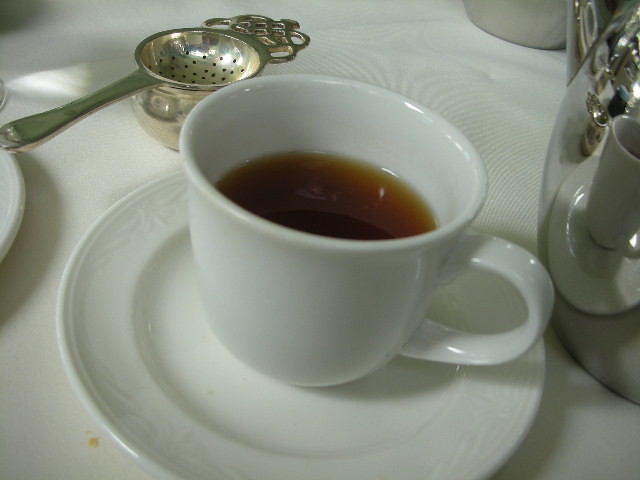This is a detailed color photograph, oriented in landscape, capturing a close-up of a white ceramic teacup filled with tea, resting on a matching saucer. The table it sits upon is covered with a pristine white tablecloth. The teacup features a tapered edge and a handle positioned to the right. Adjacent to the cup, on the left side of the table, is an ornate stainless steel tea strainer with a semi-cylindrical bowl featuring small holes, reminiscent of a colander. This strainer's holes lead into an integrated container. To the right of the cup, a shiny silver teapot is partially visible, cut off by the edge of the image. There's a minor coffee stain on the lower left corner of the tablecloth. The photo is slightly angled from the top left to the bottom right, creating a dynamic composition that emphasizes the sophisticated and serene tea setting.